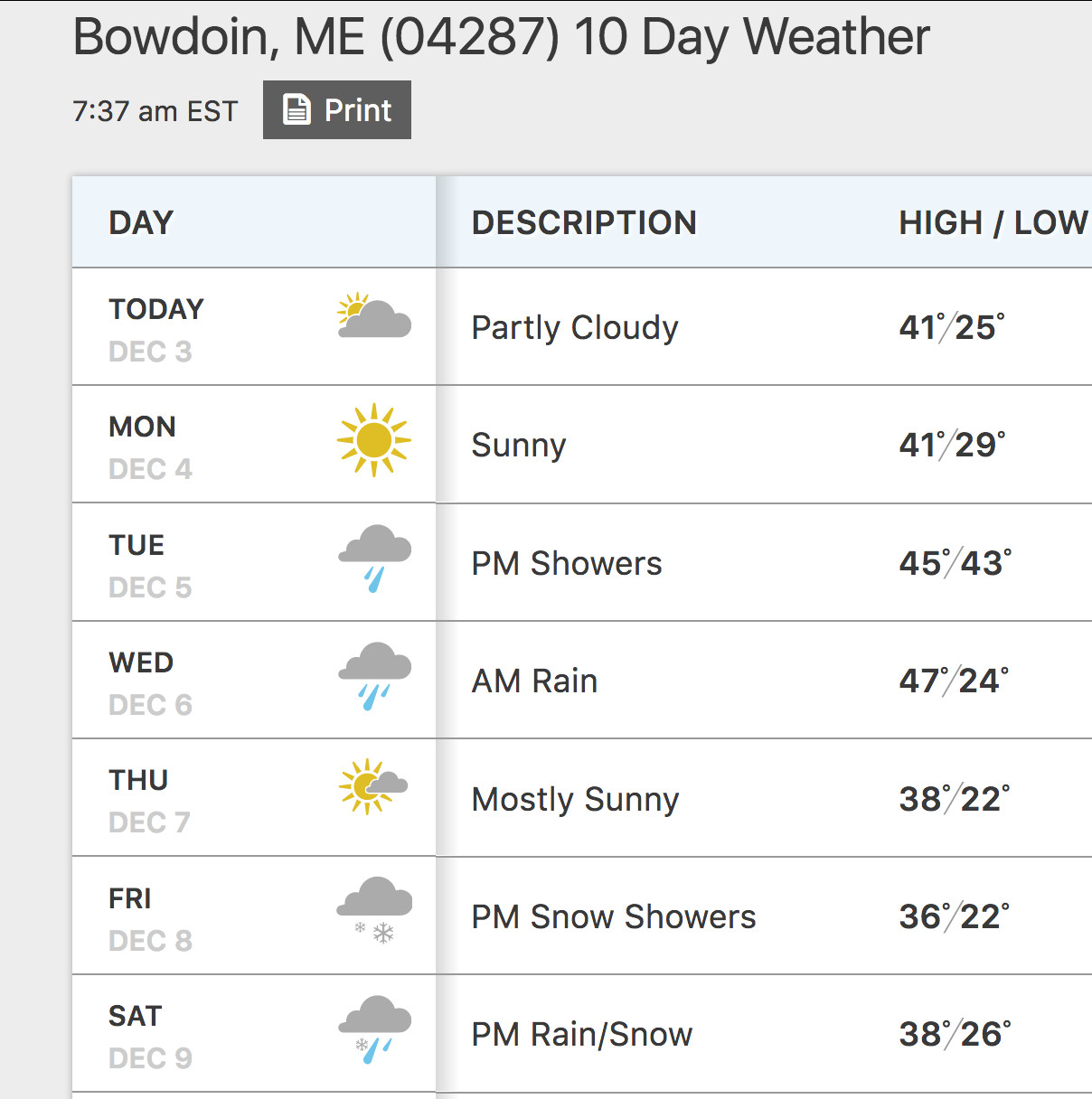This image depicts a weather application or website interface. In the top left corner, the current location is displayed as "Bodouin, M.E." with the ZIP code "04287" in parentheses. Adjacent to the location information, right-aligned, is the text "10 Day Weather" in bold black font. Below this title, the time "7:37 A.M. EST" is indicated in a smaller black font. To the immediate right, there is a gray rectangle containing the word "Print" in white text, alongside an icon of a piece of paper with a folded top-right corner.

Directly beneath this header section is a banner labeled "Day Description High/Low," presented in light blue. Following this banner is a detailed list of weather forecasts spanning from December 3rd to December 9th.

- **Today, December 3rd:** Partly cloudy, depicted with an icon of a cloud and the sun peeking out from behind it. The high is 41°F and the low is 25°F.
- **Monday, December 4th:** Sunny, represented by a sun icon. The high is 41°F and the low is 29°F.
- **Tuesday, December 5th:** P.M. showers, illustrated with a cloud and raindrops icon. The high is 45°F and the low is 43°F.
- **Wednesday, December 6th:** A.M. rain, shown with a rain cloud and droplets icon. The high is 47°F and the low is 24°F.
- **Thursday, December 7th:** Mostly sunny, indicated by a sun icon with a small cloud in front of it. The high is 38°F and the low is 22°F.
- **Friday, December 8th:** P.M. snow showers, depicted with a cloud and snowflakes icon. The high is 36°F and the low is 22°F.
- **Saturday, December 9th:** P.M. rain/snow, represented by a cloud with both water droplets and snowflakes. The high is 38°F and the low is 26°F.

This comprehensive weather forecast provides a clear and detailed outlook for the upcoming week.